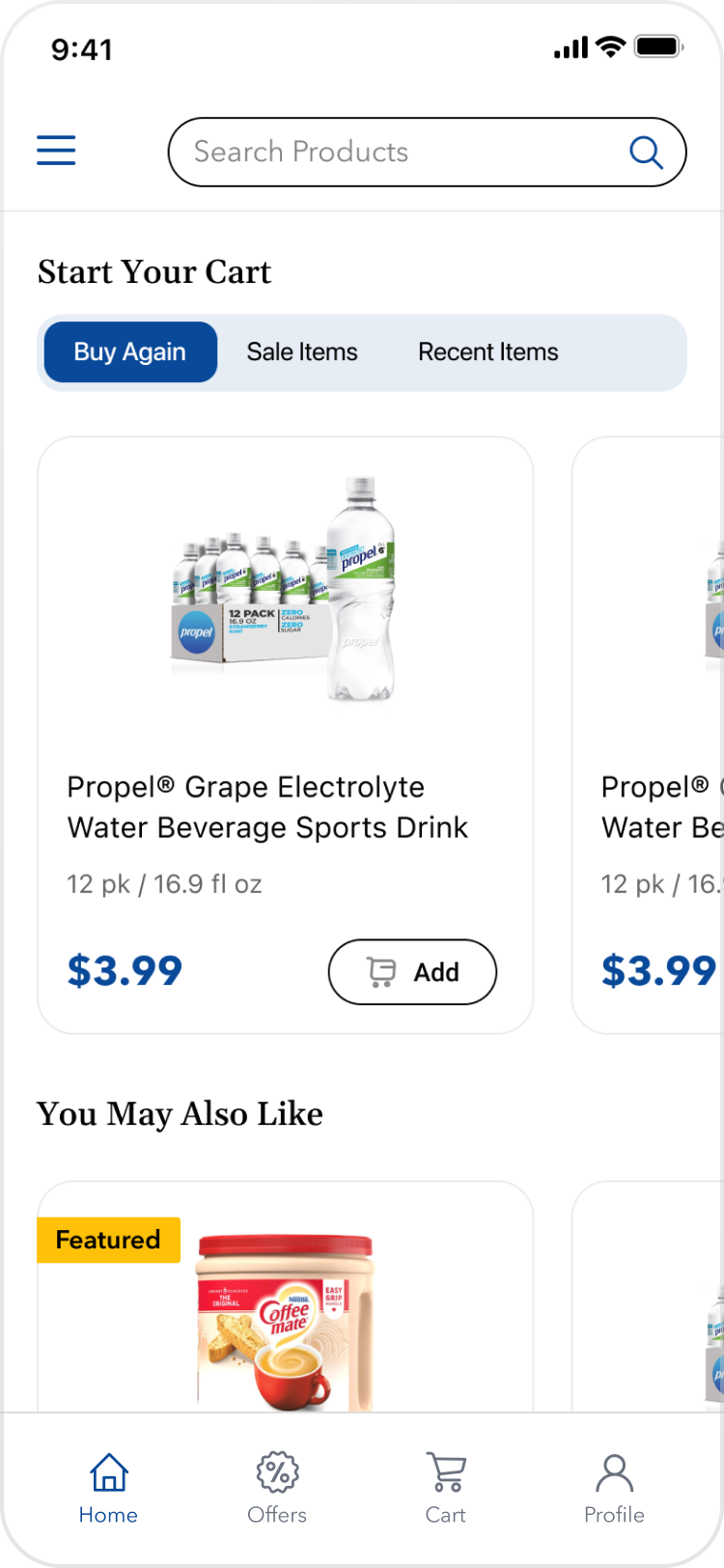This image is a screenshot of a grocery shopping app displayed on a mobile phone, featuring a predominantly white background. In the top left corner, there's a blue menu icon, and to its immediate right, a search bar with the placeholder text "search products" in light gray. Adjacent to the search bar, on the far right, is a search icon.

Beneath these elements, bold black text reads "Start your cart." Directly underneath, a long light blue bar showcases three categories: "Buy Again" on the left, "Safe Sale Items" in the center, and "Recent Items" on the right. The "Buy Again" category is highlighted in dark blue, indicating it is currently selected.

Following this, a large white box prominently displays a photo and description of a product: "Propel Grape Electrolyte Water Beverage Sports Drink." Just below this description, in small gray text, it specifies "12 pack, 16.9 fl. oz." At the box's bottom left, the price is marked as "$3.99" in large blue font. On the bottom right, there is an "Add" button.

Further down, bold black text states "You may also like," with the visible top portion of another product box, featuring a Coffee Mate creamer label, shown beneath it.

At the very bottom of the screenshot are four icons representing different sections of the app: Home, Office, Cart, and Profile.